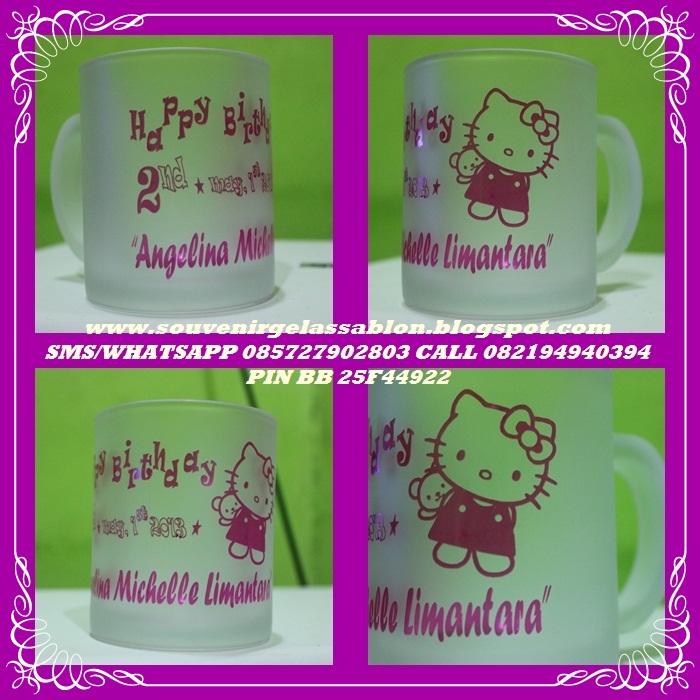In the image, there's a purple-outlined border framing four small square insets. Each inset shows a clear mug from different angles against a green background. These mugs are themed with Hello Kitty designs, featuring Hello Kitty in a dress holding a teddy bear behind her back. The mugs have white, clear-ish material and display the text "Happy Birthday, 2nd, Angelina Michelle Limanara," although the name varies between images as "Michelle Lamentara." The date "May 1st, 2013" is also visible on the mugs. Each corner of the border has swirly decorations, and a white frame surrounds the entire image. In the center, there is text displaying contact information: "www.souvernirjealassablanc.blogspot.com, SMS/WhatsApp 085727902803, call 082194940394, PIN BB25S44922."